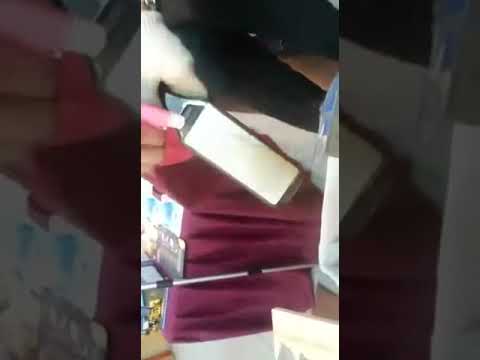The image, rotated 90 degrees counterclockwise, primarily features a vertical rectangular strip centered against black letterbox borders on both sides. The main focus is on two hands: the right hand holds a rusted, possibly curved blade resembling a machete, while the left hand, emerging from the bottom of the rotated image, appears to be steadying a gray rectangular object being cut or sharpened. The scene is somewhat blurry, but it's clear that the hands and objects are positioned on a patterned white table. Surrounding the focal objects, we see additional tools including a pair of scissors, what could be a metal file or strip, and possibly a curling iron. Toward what would be the top of the rotated image, there's a glimpse of the floor with a purple cloth draped across it, adding to the cluttered, workshop-like setting.